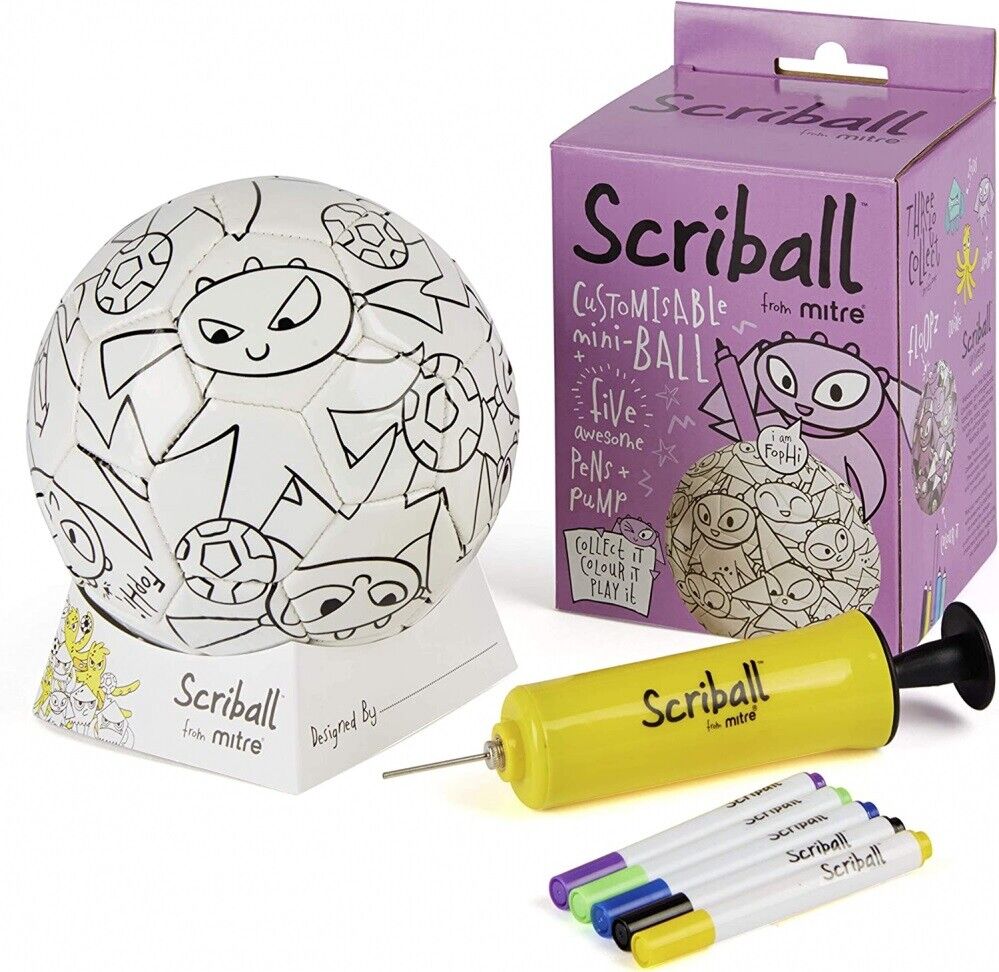The image shows a clear, brightly lit scene featuring a customizable mini soccer ball kit called "Scriball" from Mitre. The background is white, enhancing the visibility of the items. On the far left, there is a white soccer ball with black-and-white cartoon characters designed to be colored, sitting on a small white stand labeled "Scriball from Mitre" with a blank line for personalization. To the right, there is a light purple box adorned with black, white, baby blue, and yellow text and images. The box features the slogan, "Collect it, color it, play it," and includes a picture of the ball and cartoon characters. A small yellow air pump is provided, along with five markers in purple, green, blue, black, and yellow, designed for coloring the ball. The kit is marketed as a fun and creative activity, comprising all necessary components for customization and play.